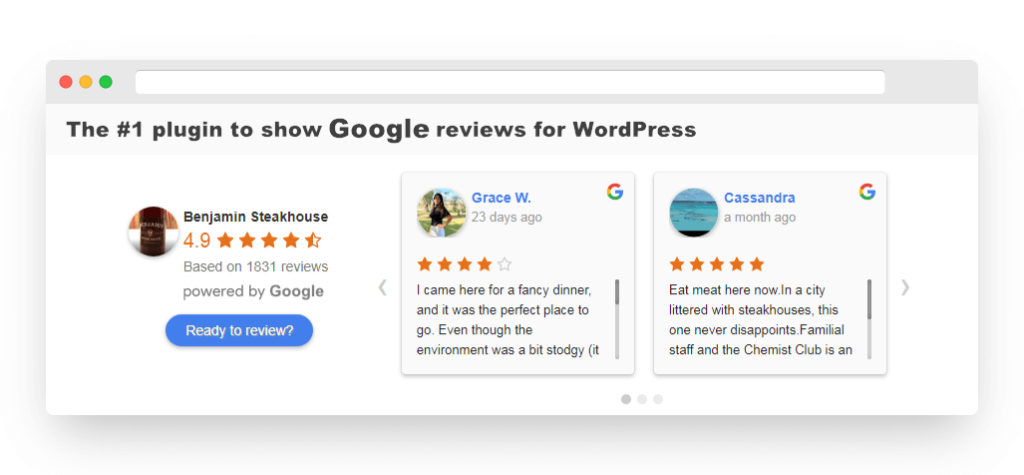### Caption:

The image showcases a detailed segment of a web page, specifically designed to display Google reviews for WordPress plugins. The layout adopts a landscape orientation and is presented in a long, narrow rectangular format.

**Top Section:**
- Across the very top of the page, there's a pale gray bar that spans the width of the image.
- Embedded within this pale gray bar is a white space, resembling a search or URL bar, where users can input text. Despite its appearance, it lacks a dedicated search icon.
- Situated to the left of this bar are three horizontal dots colored red, yellow, and green, respectively.

**Main Content:**
Below the gray bar, the main content section appears, featuring a white background. Aligned to the left within this white section, bold black text announces: 
- "The #1 plug-in to show Google reviews for WordPress," where the word "Google" is rendered in a larger font size than the surrounding text.

**User Reviews:**
Beneath this headline are three user reviews, organized in a horizontal row:
1. **Left Review (No Outline):**
   - Title: "Benjamin's Steakhouse"
   - Rating: 4.9 out of 5 stars, depicted with four and a half yellow stars.
   - Additional Info: A small user profile circle, possibly featuring a beer can icon. The text notes the rating is "based on 1831 reviews powered by Google."
   - Action: A blue oval button labeled "Ready to review?"

2. **Middle Review (Pale Gray Outline):**
   - User: "Grace W.," with her name in small bold blue font. A profile picture shows her outdoors.
   - Timestamp: "23 days ago"
   - Rating: 4 out of 5 stars
   - Review Text: "I came here for a fancy dinner and it was a perfect place to go even though the environment was a bit stodgy. (It..." followed by a vertical scroll bar, indicating additional text.
   - Icon: The multicolored Google "G" logo in the upper right corner.

3. **Right Review (Pale Gray Outline):**
   - User: "Cassandra," with her name also in bold blue font. A bluish profile picture is displayed.
   - Timestamp: "A month ago"
   - Rating: 5 out of 5 stars
   - Review Text: "Eat meat here. Now, in a city littered with steakhouses, this one never disappoints. Familial staff and the Chemist Club..." (Note: 'Chemist Club' is capitalized), followed by a scroll bar for more text.

**Navigation:**
- On the very right edge of the image, a right arrow is visible, allowing users to navigate through additional reviews.

The design emphasizes user-generated feedback and features interactive elements such as scroll bars and clickable buttons, enhancing user experience.